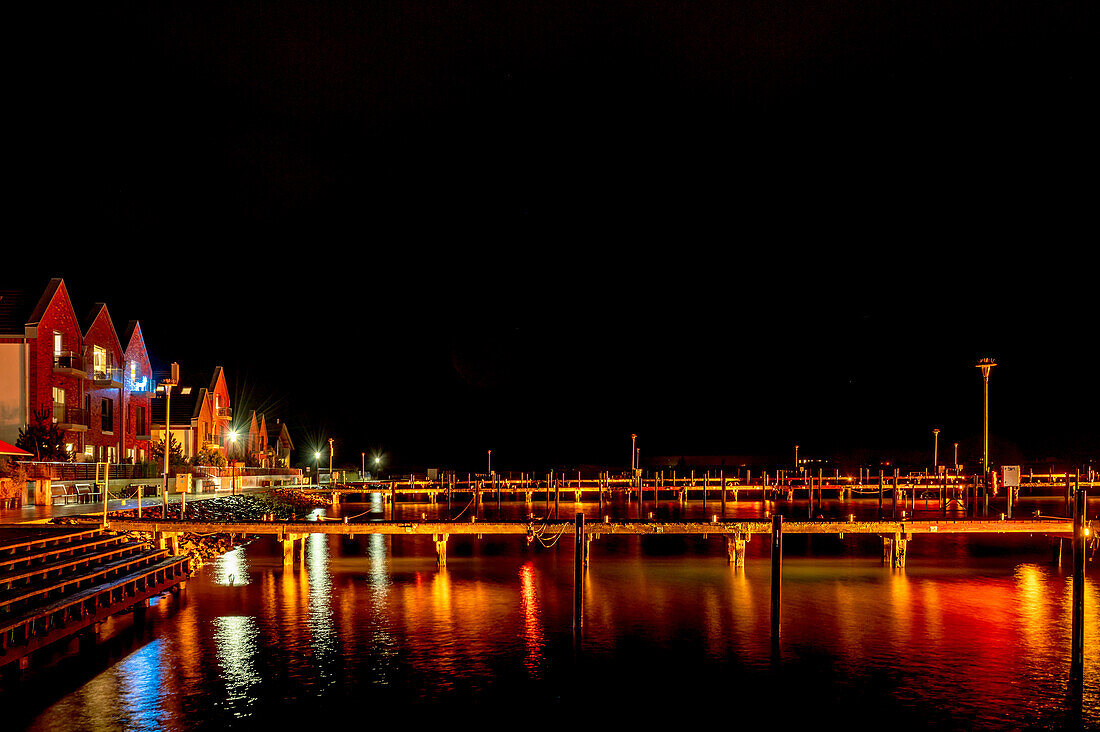This photograph captures a tranquil nighttime scene in a harbor town. Dominated by a pitch-black sky devoid of stars or the moon, the image is primarily shadowed, save for the bottom third where the harbor comes into view. The docks are empty of boats and people, lending an eerie calmness to the scene. On the left side of the image, dockside buildings with pointy roofs are illuminated by various internal lights, casting an inviting red, orange, and yellow glow. These lights create vivid reflections on the water's surface, enhancing the picturesque quality of the scene. Additionally, lampposts lining the street between the docks and the buildings further light up the area, and a set of stairs on the left descends toward the water, adding an element of depth to the tranquil, yet vividly lit harbor scene.